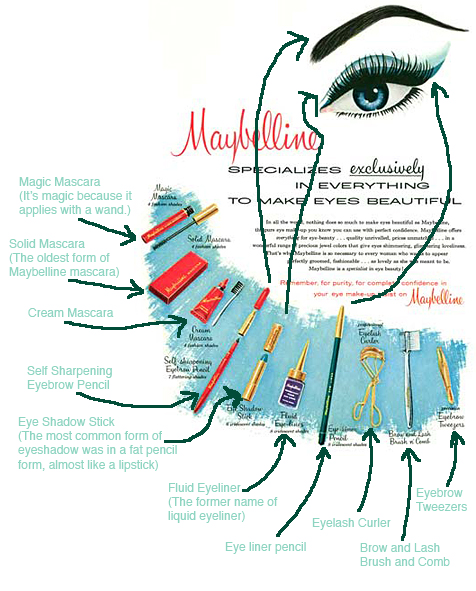This illustration appears to be an older, possibly 1960s, advertisement for Maybelline, centered on their eye makeup products. At the top, it features a detailed, artistic rendering of a woman's eye with blue eyeshadow styled in a wing shape, long black curled lashes coated in mascara, and a similarly wing-shaped black eyebrow. Underneath this central image, "Maybelline" is prominently displayed in large red cursive letters, accompanied by the slogan "specializes exclusively in everything to make eyes beautiful." 

Beneath the text lies a blue background layer which displays various meticulously detailed drawings of eye makeup products. Each product image is annotated with arrows pointing to corresponding labels and descriptions. Featured items include several types of mascara such as "magic mascara" (applies with a wand), "solid mascara" (the oldest form, housed in a red box), and "cream mascara" (in a red tube with a small brush). The assortment also showcases an "eyeshadow stick," "self-sharpening eyebrow pencil," "fluid eyeliner" (previously known as liquid eyeliner), "eyeliner pencil" (a green pencil), "gold eyelash curler," "brow and lash brush and comb" (a silver tool), and "eyebrow tweezers" (in gold).

Additional text within the advertisement, though largely too small to read, reinforces the theme of Maybelline's dedication to purity and confidence in eye makeup products. The detailed annotations and arrows not only highlight each product but also demonstrate where and how each item is applied, creating an informative and visually engaging promotional piece.